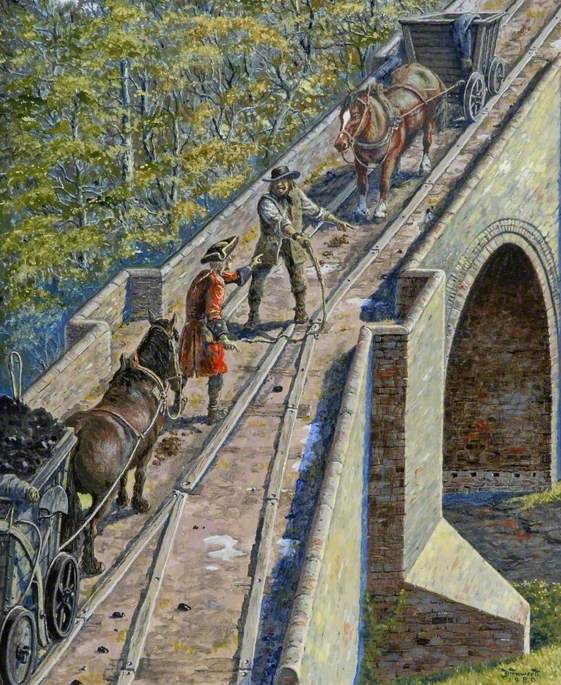The image portrays a historically themed painting from the early 19th century, set on an arched stone bridge that spans a creek below. The bridge is constructed from cinder blocks and features a large opening to allow for passage underneath. There are trees in the top left corner, and some shrubbery is visible beneath and around the bridge.

On the bridge, two men confront each other head-on in an intense standoff. The man on the left is dressed in a red coat trimmed in black, black boots, and a black cap with gold trim, resembling a uniform from the Civil War era. He is leading a horse that pulls a cart filled with black material, likely coal, accompanied by a gray shovel attached to the side. 

Facing him is a man who looks like a cowboy, wearing a black Stetson hat, a green vest over a white shirt, and brown pants. His cart appears empty but has what looks like a folded jacket draped over it. Both men are animated, each pointing fingers and clutching whips, seemingly locked in an argument about who should have the right of way. This confrontation, set against the backdrop of the old bridge and the timeless costumes, creates a vivid depiction of a historical clash.